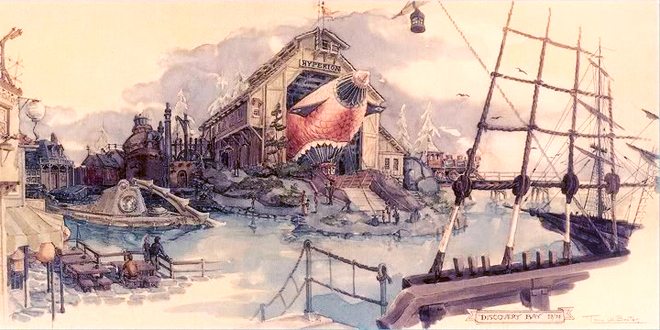The image is a detailed, watercolor-style illustration of a small town set in a steampunk-inspired, fantasy world. Central to the image is a large, reddish-orange structure labeled "Hyperon." This structure resembles a blimp or rocket ship with a scaly design, black wing-like appendages, and additional black details at the bottom and points. The blimp appears to be emerging from a hangar with stairs extending from its front. The setting around it features cobblestone streets and seafaring ships, including an old-fashioned pirate ship and a steampunk submarine-like vessel on the left. The background, characterized by muted colors such as yellows, light blues, purples, and reds, fades into a sky filled with clouds, giving the entire scene a nostalgic, retro atmosphere. Below the central structure, there is a significant white space resembling netting, and towards the bottom, the title "Discovery Bay" can be seen, suggesting the town's name. The overall palette of the illustration remains subdued, with predominant browns, enhancing its vintage, alternate history aesthetic.